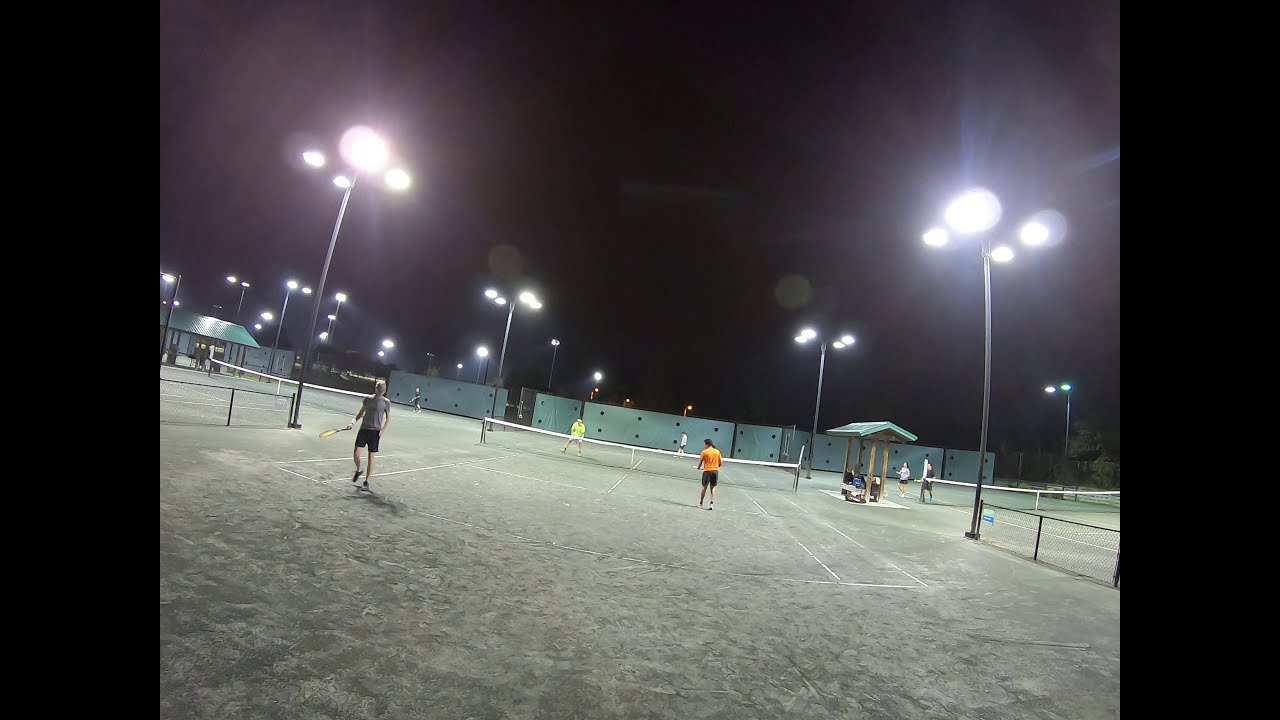This nighttime photograph captures a bustling scene at a tennis complex featuring three courts. The central focus is on a doubles match taking place on a weathered, textured court, likely paved, although it has been mistaken for grass by some due to its green appearance. The court lines are worn and modeled, consistent with the court's rough surface. Two players on each side are engaged in the match, with one player facing the camera and the other with their back towards it, poised for a serve. The image is taken with a wide-angle lens, making the scene appear more expansive. Bright lights from multiple street lamps illuminate the courts, casting a stark contrast against the pitch-black sky. In the background, a green partition wall encloses the area. Additional players are seen practicing or warming up on adjacent courts, adding to the competitive and lively atmosphere of the scene. Observers are sparsely distributed around the area, possibly indicating the presence of more intense games elsewhere within the complex.